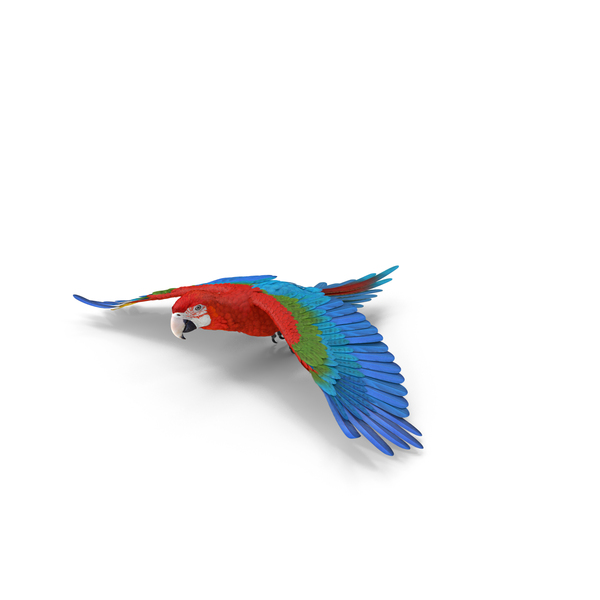This image showcases a close-up view of a vibrant parrot in flight against a white background, making it appear potentially computer-generated. The parrot, displayed in an outdoor setting, has a striking red head and body, transitioning to green feathers where the wings extend outward. Further along the wings, the green blends into turquoise, which deepens into a darker blue with a hint of purplish blue towards the tips. The tail is predominantly blue with a prominent red stripe. The bird features a predominantly white beak with some black elements near the eye area. The parrot's wing points toward the top right corner, and its head is inclined toward the top left corner. A distinct shadow cast by the parrot adds depth to the overall composition.